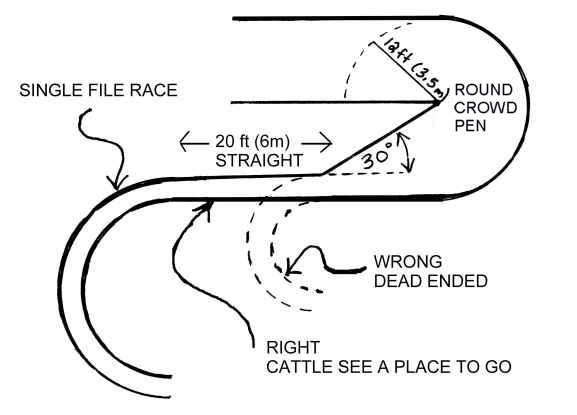The black and white diagram illustrates the setup of a cattle pen with intricate labeling and a focus on animal movement. At the top of the image is a curved path leading to the right with a label that reads "round crowd pen" indicating a radius of 12 feet (3.5 meters) and an angle of 30 degrees. Another curve branches off to the left but ends abruptly. A straight line extends from the round crowd pen with the label "20 feet (6 meters) straight." Along this path, various labels guide the viewer: "single file race" (describing the narrow pathway), "wrong, dead ended" (indicating an incorrect route), and "right, cattle see a place to go" (marking the correct path for cattle movement). The overall shape resembles a backwards 'S,' with text primarily on the right side of the diagram detailing every segment. This diagram appears to serve an educational purpose, explaining the design elements of an effective cattle pen.